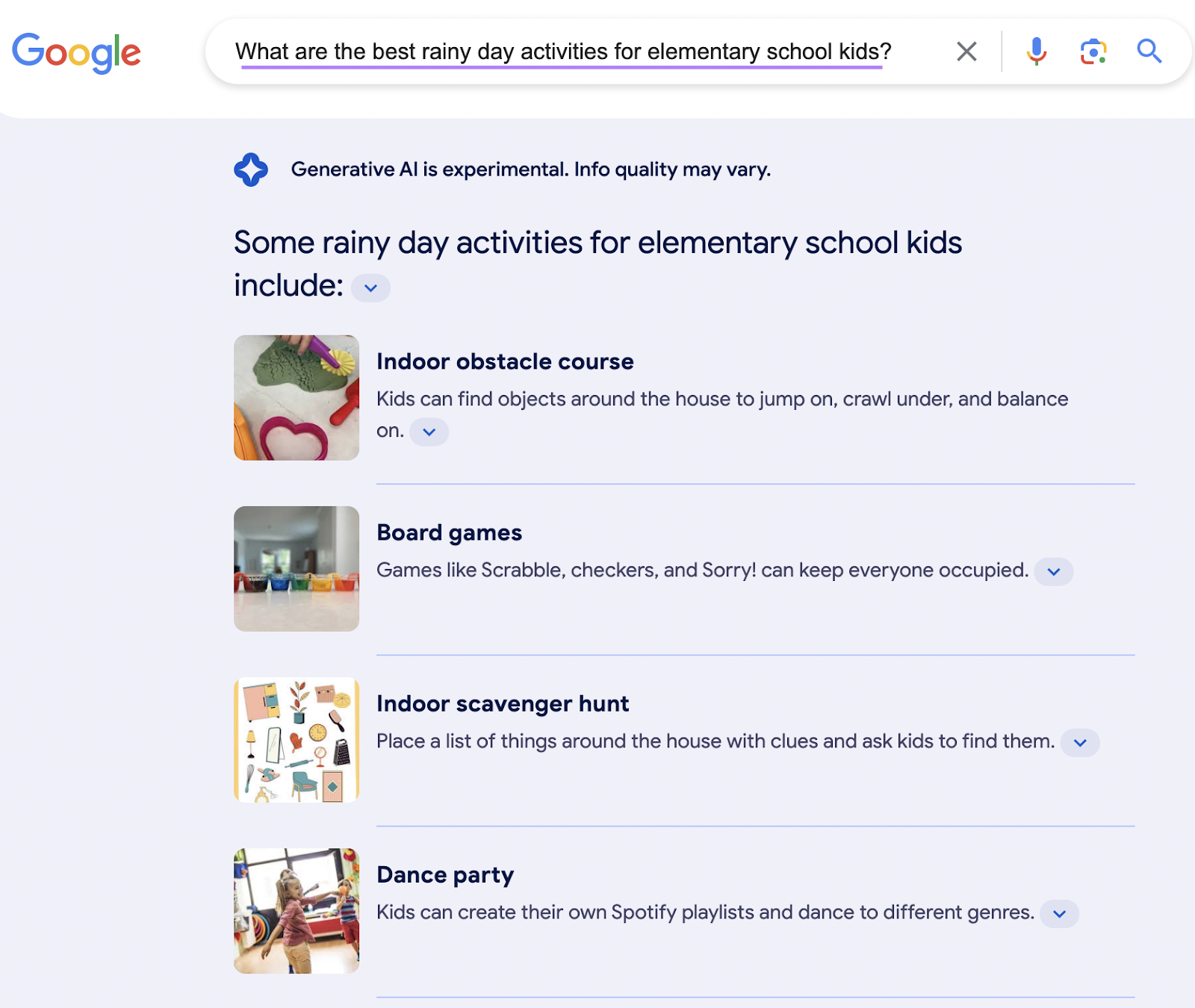The image displays a printed page from a Google search result. The Google logo is prominently positioned on the top left. The search query, "What are the best rainy day activities for elementary school kids?" follows next to the logo. To the right of the query, there are icons including a microphone, an hourglass, and another unspecified symbol.

Centered below the search bar, there is a section header stating, "Generative AI is experimental. Info quality may vary." This indicates that the following content is generated by experimental AI and may not be completely accurate.

The main content comprises a list of suggested rainy day activities for elementary school kids:

1. **Indoor Obstacle Course**: Children can use household items to create obstacles to jump over, crawl under, and balance on.
   
2. **Board Games**: Classic games like Scrabble, Checkers, and Sorry can engage the entire household.
   
3. **Indoor Scavenger Hunt**: A game where kids search for items around the house based on a provided list and clues.
   
4. **Dance Party**: Kids can curate their own Spotify playlist and dance to various music genres.

To the left of each activity description, there are illustrative photos showing examples of these activities. The text and images provide a comprehensive guide for organizing fun indoor activities for children on rainy days.